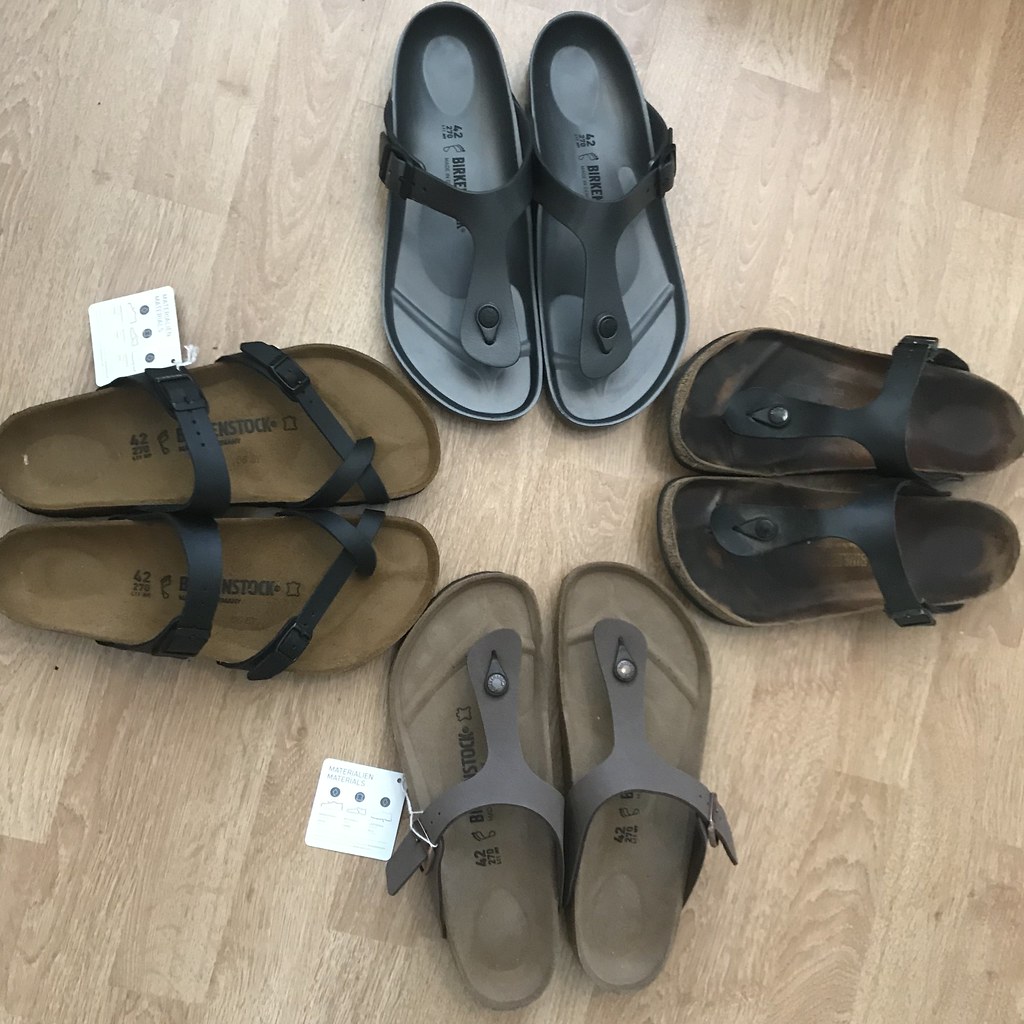This is a detailed top-down photograph depicting four pairs of Birkenstocks arranged in a cross formation on a light brown wooden laminate floor. The toes of each pair point inward, forming a small square of floor at the center. The Birkenstocks vary in condition; one pair is visibly worn with significantly darkened soles, indicating extensive use. Two pairs feature white tags, suggesting they are new or for sale, although one of these tagged pairs shows some wear with visible toe prints. The pairs include different materials: the black pairs appear to be plastic, while the brown pairs are made of leather. The bottom pair has light brown straps, and the left pair has dark brown straps, both adorned with white tags. The right pair, darker with black straps, and the top pair, gray with black straps, complete the collection. The lighting appears artificial, illuminating the arrangement and emphasizing the contrast between the new and worn footwear.